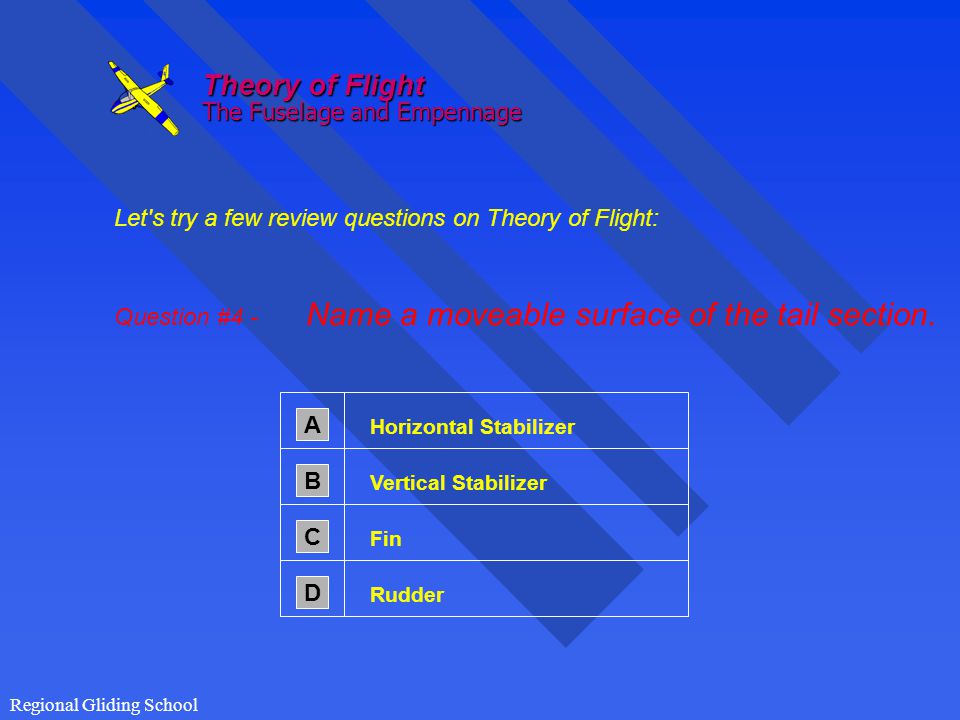This image features a slide from an instructional manual with a blue background and some streaks. At the top, bold red text reads "Theory of Flight," followed by "The Fuselage" and "Empennage" (spelled E-M-P-E-N-N-A-G-E). To the left, there is a small graphic of a yellow and blue airplane. Below, in yellow letters, it says, "Let's try a few review questions on Theory of Flight." The slide specifically addresses question number four, which asks, "Name a movable surface of the tail section," highlighted in red. Four multiple-choice answers are listed with gray squares: A. Horizontal Stabilizer, B. Vertical Stabilizer, C. Fin, and D. Rudder (R-U-D-D-E-R). The image appears to be a part of the Regional Lighting School curriculum.